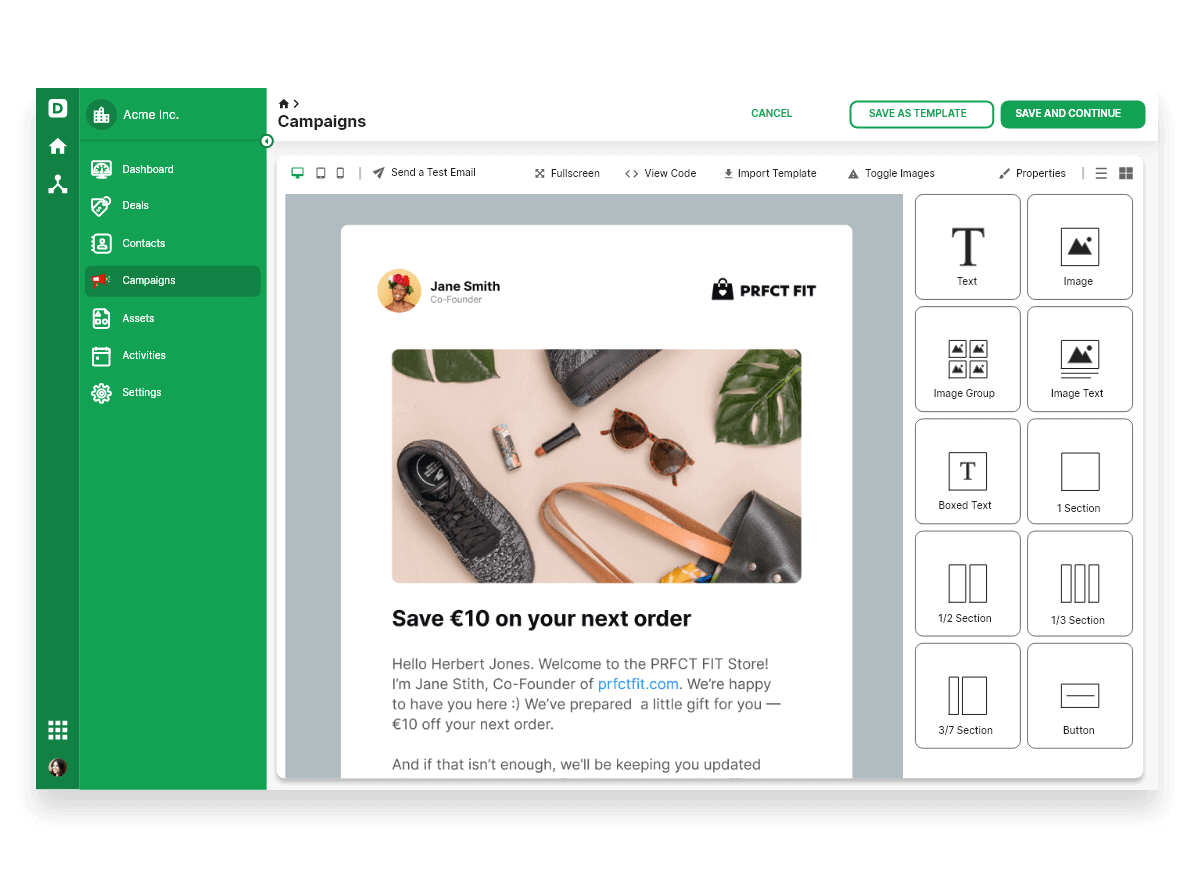The image depicts a screenshot of a computer interface. On the left side, there is a narrow dark green sidebar hosting five icons—three at the top and two at the bottom. The bottommost icon appears to be a circle containing a profile picture. Adjacent to this is a wider light green sidebar that features a small border at the top. This top section includes an icon and some text, followed by seven additional icons each accompanied by a title. 

Dominating the remaining portion of the screenshot is a white background. Across the top of this section, a white border features the word "Campaign," with two command buttons: "Cancel" in green and a white button labeled "Save as a Template." There is also a green button that reads "Save and Continue."

Beneath this top section, another white bar runs horizontally across the screen, populated with several small, indistinguishable icons and text labels. A larger green square is positioned below this bar on one side. Inside the green square is a white rectangle that displays the name “Jane Smith” alongside a profile picture located to the left. Additionally, the image showcases a variety of items including shoes, glasses, a purse, and a leaf, accompanied by the text "Save 10 euros on your next order."